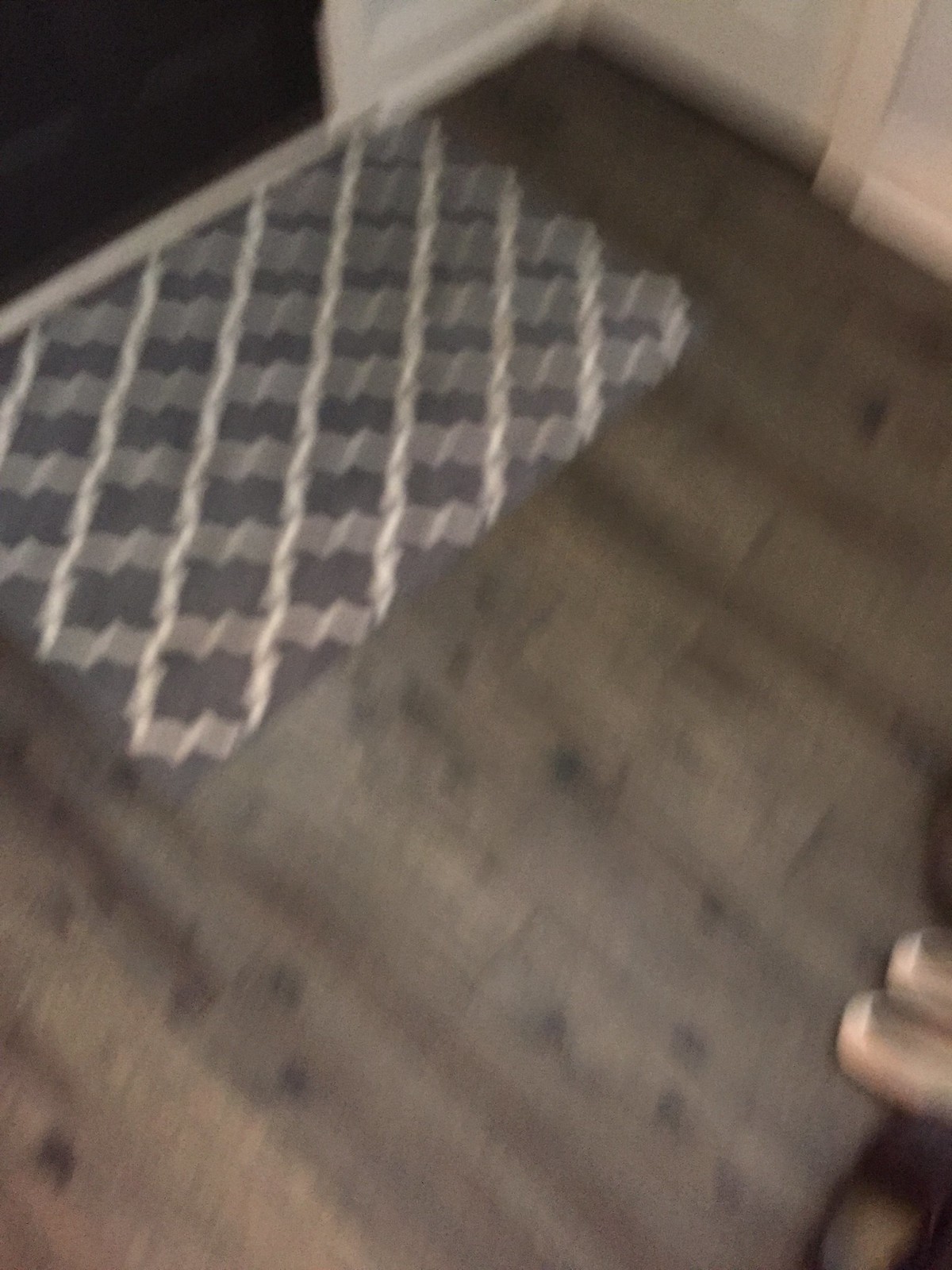The photograph is an extremely blurred image of a doormat on a wooden porch or stoop, viewed from above. The porch is rustic with visible knot holes and scuff marks, indicating wear. The wood is predominantly brown. In the upper left-hand corner, there is a brown door partially visible along with the white threshold. Adjacent to the door is a doormat featuring a complex pattern of white crisscrossing wavy lines and thicker gray squiggly lines on a dark gray background. Below and to the right of the mat, the image reveals a pair of pink shoes, potentially ballet slippers, along with some indistinct brown objects. The perspective suggests an intimate, everyday scene, possibly at the entrance of a home, where the welcoming mat ties together a rustic and homey aesthetic.